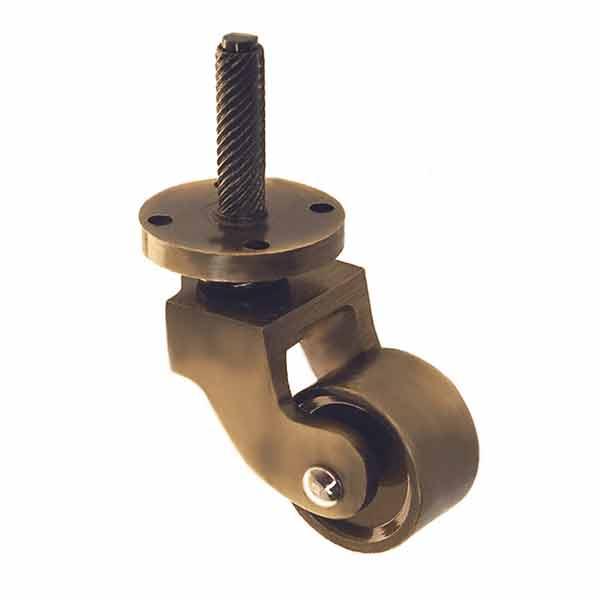The image showcases an extreme close-up of a bronze-colored wheel attachment set against a white background. The wheel, placed to the right of the photo, features a smooth texture and a reflective silver screw linking it to a square-shaped swivel. Emerging centrally from the swivel is a spiraling spoke designed for secure attachment to items like furniture, rolling carts, or drawers. The base of the spoke area includes four additional holes, presumably for reinforcement screws, ensuring sturdy installation. The detailed view highlights the functional design of this wheel meant to facilitate the mobility of various products.